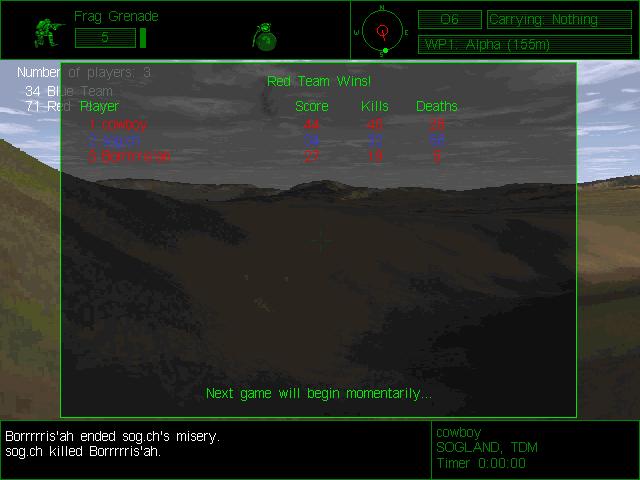The image presents a square-shaped digital screen, suggesting it is from a game interface. The bottom left of the screen displays several lines of white text. The first line reads "BORRRRRISAH" followed by "end it", "SOG.CHS", and "misery". Directly beneath these words, the text states "SOG.CH killed BORRRRRISAH". The repetition and varied spacing of "BORRRRRISAH" appear to emphasize a dramatic or significant event within the game. Furthermore, centralized on the bottom left corner, the screen displays the word "cowboy". Below this, the text "SOGLAND, T-V-M" is visible, likely referring to a location or a player name. The bottom-most line of text presents "timer" followed by "zero", possibly indicating that either a countdown has ended or that no time limit remains. Overall, the image's text suggests the conclusion of an in-game event, laden with impactful elements and player interactions.